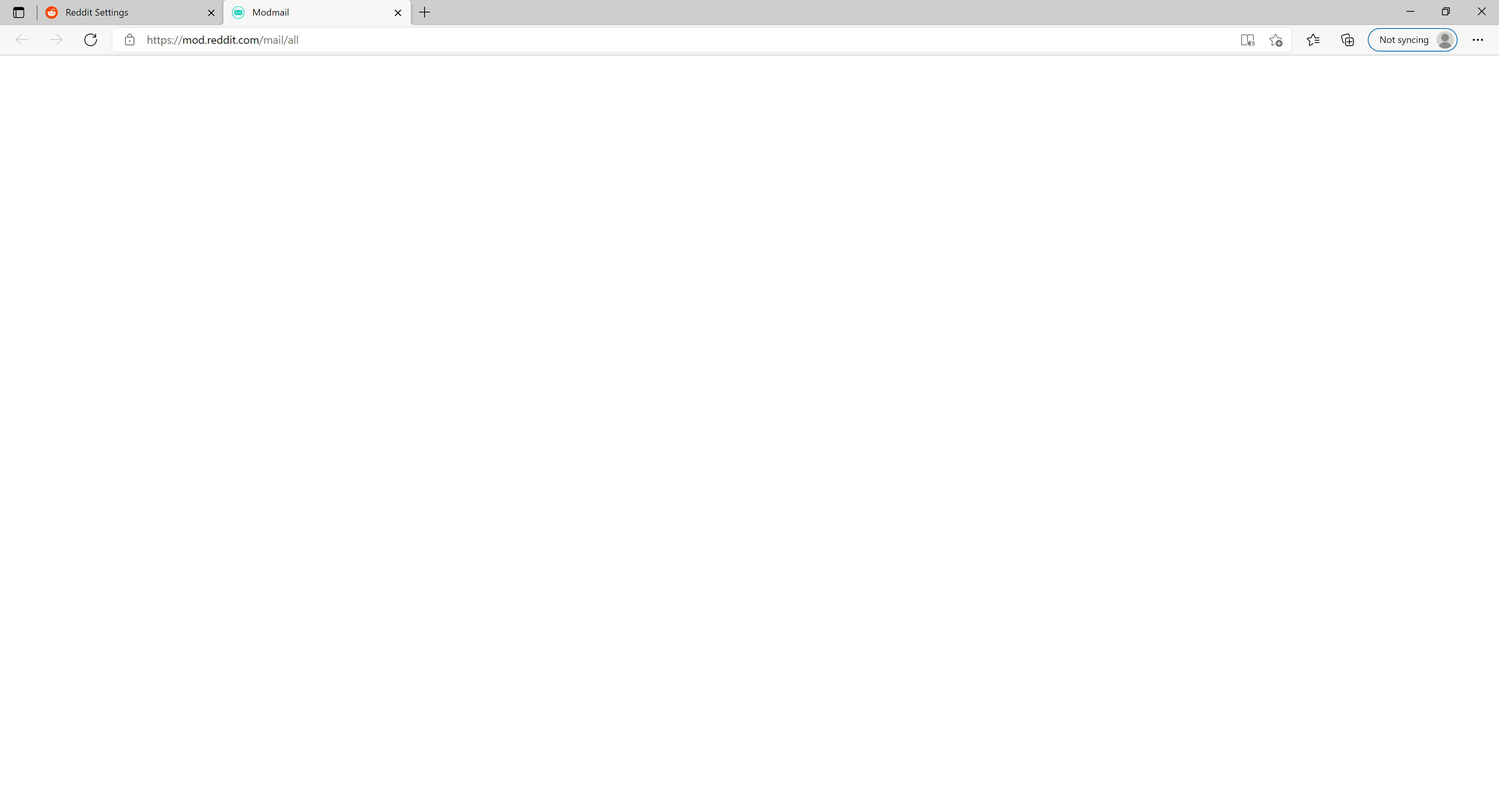The image showcases a desktop version of a web browser, likely Internet Explorer, with a focus on a tab titled "Mod Mail." This is the second tab the user has opened, as indicated by its position. Another visible tab is labeled "Reddit Settings" and features the Reddit logo in the top header. The interface includes typical browser controls such as options to close, minimize, or entirely remove the tab from view without fully closing the browser.

The URL bar shows the address "https://mod.reddit.com/mail/all," but the content area is a blank, white screen, suggesting that the actual website hasn't loaded properly. The browser's forward and back buttons near the URL are grayed out, indicating they are inactive. Only the refresh button appears functional.

Additionally, there is a bookmark icon visible on the toolbar. The browser displays a notification in the header that the profile is not syncing, with a blank profile photo next to this message. There is also an ellipsis (three dots) button, which, when clicked, likely provides access to various browser settings and options for interacting with the website.